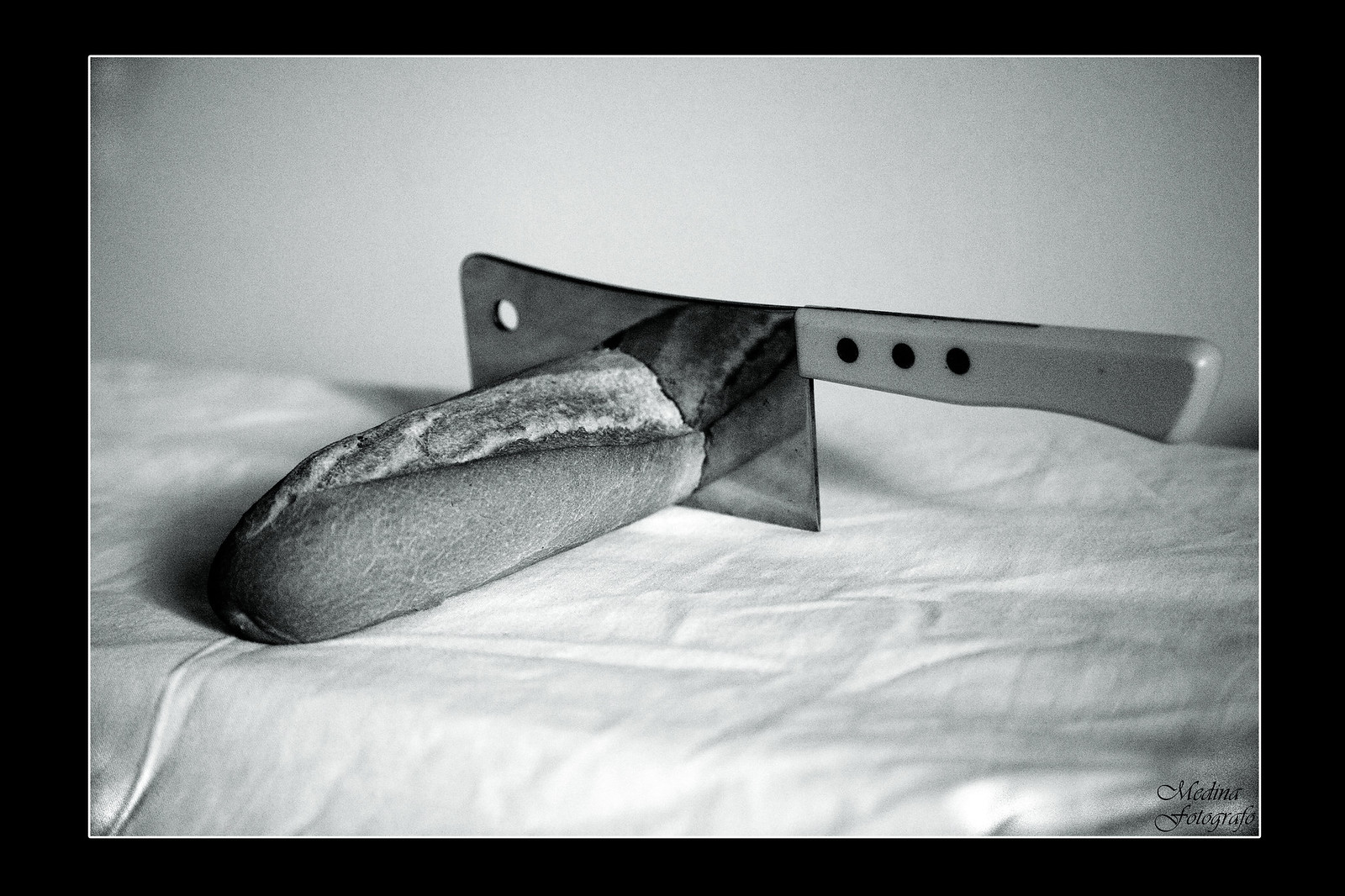This is a highly detailed black-and-white photograph with an artistic touch, framed by a solid black border with a thin white outline. The central focus of the image is a butcher's cleaver cutting through a six-inch portion of a baguette. The cleaver, positioned upright, rests against the bread on a white linen or tablecloth, though no hands are visible. The blade features a hole in the top left corner, typical of a butcher's cleaver, and it captures the reflection of the baguette. The bottom right corner of the photograph is signed with the name "Medina Fotografo."